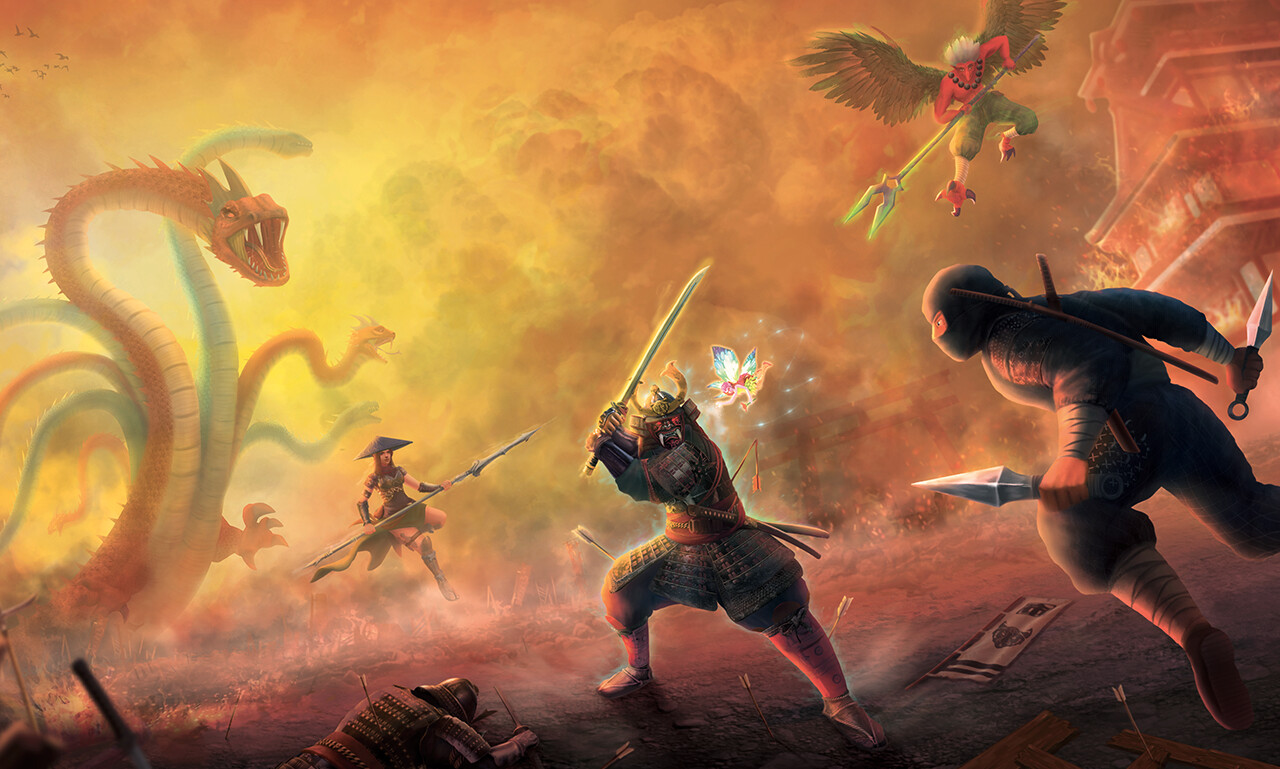The image is a highly detailed fantasy illustration depicting an intense battle scene. Central in the image is a formidable samurai clad in black armor with red garments beneath, featuring red eyes and golden horns extending from his head. He wields a large sword and stands steadfast, confronting a menacing ninja dressed in all black with a mask, who brandishes two silver knives and appears to be lunging towards the samurai. To the left, a massive, multi-headed dragon serpent with heads colored in hues of green and red, each set of eyes blazing and fangs bared, looms intimidatingly. Smoke and vibrant fumes fill the air, adding chaos to the scene. Above, an angelic warrior with red plumage and white wings hovers, gripping a blue spear as if poised to strike. The background is alive with additional warriors, some armed with spears, forlorn flags waving amidst the turmoil, fallen fighters, and a decaying landscape suggesting devastation. The colors of the artwork are dramatic and intense, dominated by black, purple, blue, red, yellow, and orange, with an ominous building shadowing the background. This dynamic illustration captures a climactic moment in a fantastical warrior saga.